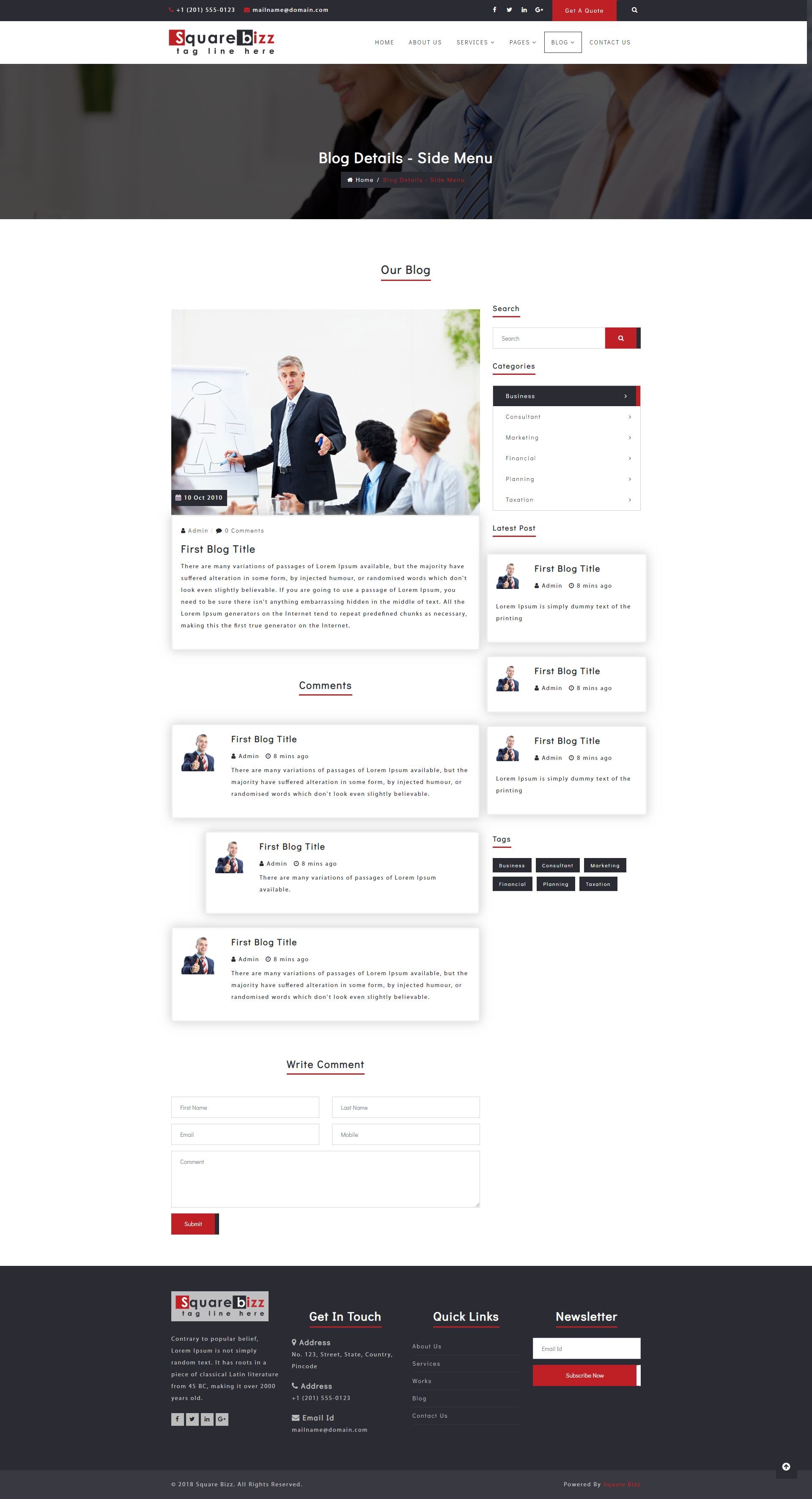Here is a detailed and cleaned-up caption for the image described:

---

The homepage of the website "Square Biz" (stylized as "Square B-I-Z-Z") features a professional interface with a tagline prominently displayed. At the top, there is a visible phone number for contact, along with an email option. Users can connect with the business through various social media platforms including Facebook, Twitter, Instagram (represented by "IN"), and Google Plus. There is also a feature to request quotes directly from the website. The navigation bar includes buttons for "Home," "About," "Services" (with a dropdown menu), "Pages" (with a dropdown menu), "Blog," and "Contact Us."

Beneath the navigation bar, there is an image of four business professionals: three men in different-colored dress shirts and ties, and a woman in a business suit with a dress shirt and tie, positioned on the far left. Below this image, the section titled "Our Blog" is marked in black with a red underline. The first blog entry, dated October 10th and authored by the admin, features a man presenting a flow chart to an audience, alongside a comments section for visitor engagement.

To the right of the blog, a search function is available. Below this are various categories for blog posts including "Business," "Consulting," "Marketing," "Financial Planning," and "Taxation." Tags related to different topics are listed for user convenience, and visitors are encouraged to leave comments by filling out a form with their first and last name, email, mobile number, and comment, followed by a submit button.

At the top of the webpage, there are links for "Get in Touch" and "Quick Links." Additionally, users can subscribe to a newsletter by entering their email address.